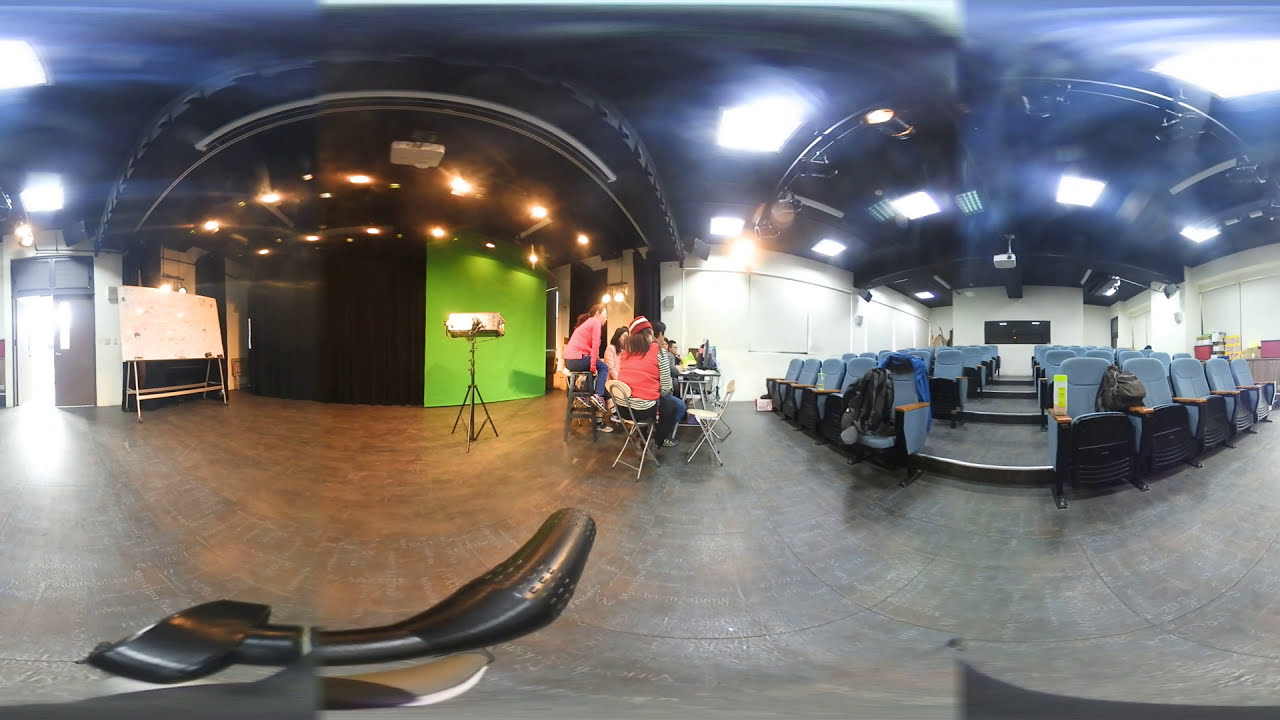This panoramic fisheye photograph captures a small auditorium or classroom-like space set up for a theater rehearsal. The image features blue, cushioned theater seats on the right side, mostly unoccupied and some with backpacks, suggesting a school setting. Center and left of the frame showcase a stage area with a few casually dressed actors in jeans, seated on a mix of metal chairs and stools. The actors wear a variety of casual clothing, including red and pinkish shirts, and one person at the forefront has a vest and a neck cap. A green wall serves as the stage backdrop, accompanied by a whiteboard on an easel. Overhead, white fluorescent lights illuminate the space, which also features a black ceiling and a white back wall. To the far left, a gray double door with one side open lets in a beam of light. Visible in the lower left corner are parts of camera equipment, hinting at a recording setup. The overall scene, devoid of audience members, underscores the rehearsal atmosphere.